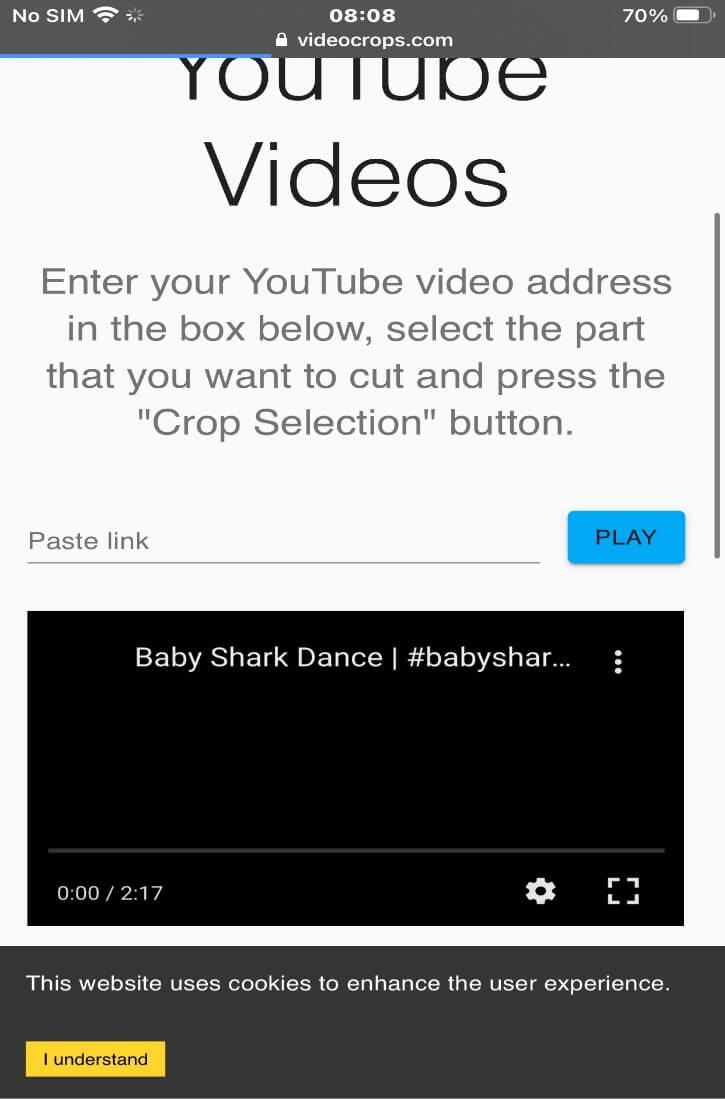This is a detailed screenshot captured from a cell phone displaying a YouTube video screen. The phone's status bar at the top is black, indicating "No SIM" on the left and showing a Wi-Fi connection icon. In the center, the time reads 8:08, and beneath it, there's a white lock icon next to the website address "videocrops.com." On the right side of the status bar, the battery capacity is displayed at 70% alongside the battery icon.

Beneath the status bar, there are three distinct sections. The top section is light gray with black and light gray text. At the very top of this section, it reads "YouTube videos," followed by a light gray description: "Enter your YouTube video address in the box below. Select the part that you want to cut, and press the crop selection button." Below this description, there is a field labeled 'Paste link,' accompanied by a blue button labeled 'Play' on its right.

Directly beneath this section, a video has been selected within a black box. The video's title at the top is "Baby Shark Dance #babyshark," with three vertical white dots to the side. At the bottom of this black box, the video duration is indicated as "2:17." To the right, there's a gear icon for settings and a box outline for expanding the video.

The final section at the bottom is gray, containing a message: "This website uses cookies to enhance the user experience." In the lower left corner, there's a yellow button labeled "I understand."